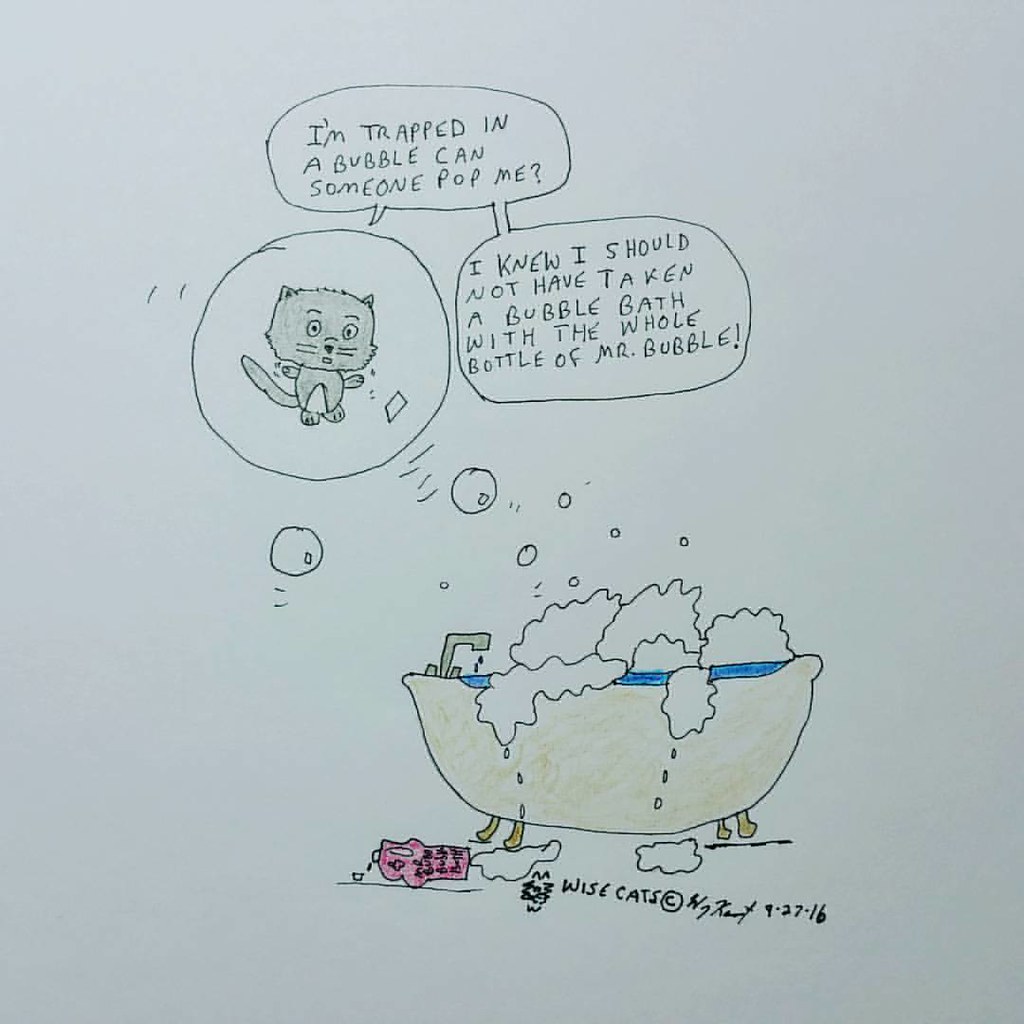The image is a hand-drawn illustration on a piece of white paper, likely done with an ink pen and crayons. At the top, there's a gray cat figure encased in a bubble with a thought bubble that reads, "I'm trapped in a bubble, can someone pop me? I knew I should not have taken a bubble bath with the whole bottle of Mr. Bubbles!" Beneath this, the text says, "Wise Cats," followed by a copyright and a signature dated 9-27-16. Below the text is a detailed drawing of a yellow, claw-foot bathtub overflowing with white foam and water, with bubbles floating above. There's a pink bottle marked as Mr. Bubble spilling onto the ground next to the tub.